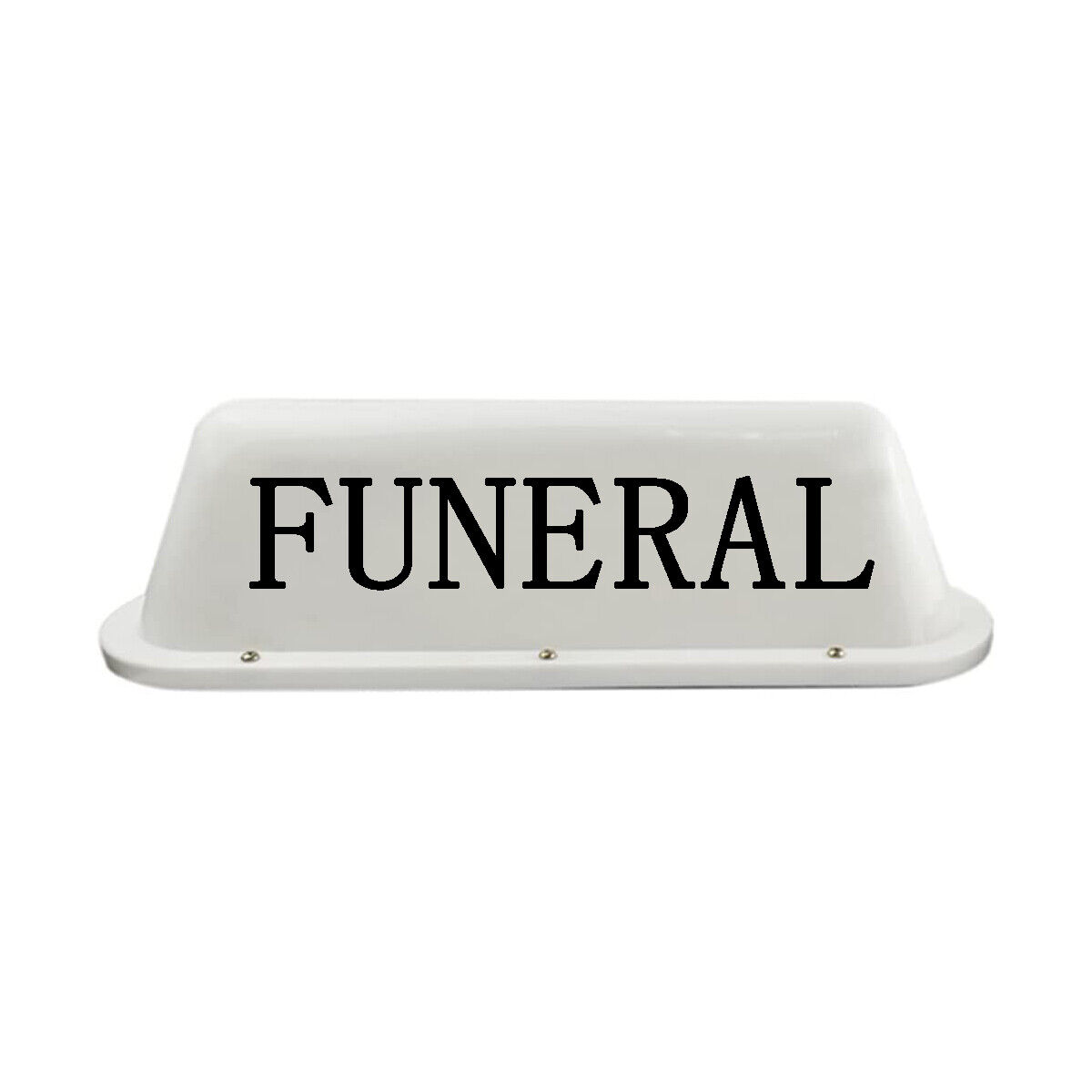The image features a white, shiny sign shaped like an upside-down bathtub, resembling a ceramic butter dish. It has a hollow, oval base that tapers and rounds off at the top. Bold black serif letters spell out "FUNERAL" prominently on the sign, centered on its surface. The sign also features three screws on the front, likely for attachment to the top of a vehicle, suggesting it is used for funeral processions. The background is a pure white, emphasizing the sign's details and its function as a vehicle-mounted indicator for funerals.